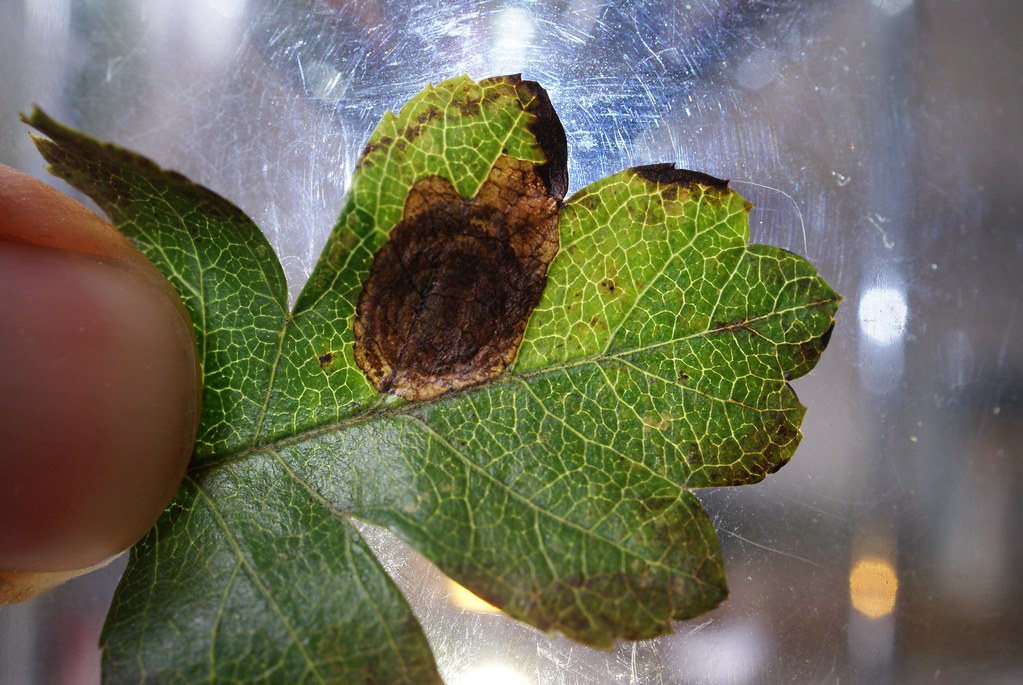In this detailed close-up image, a person holds a small green leaf between their thumb and index finger. The leaf prominently features a large, irregularly shaped brown burn mark in its center, with additional browning along some edges, suggesting it may have been partially burned using a magnifying glass or similar tool. Visible on the leaf are intricate yellow veins that stem from the center and extend outward. The background includes a scratched, somewhat opaque glass, giving a grayish tint with hints of blue at the top, and a light source shines through the leaf, highlighting its detailed structure. The overall image captures the delicate interplay of light and texture, emphasizing the fine details of the leaf's anatomy and the effects of the burn mark.